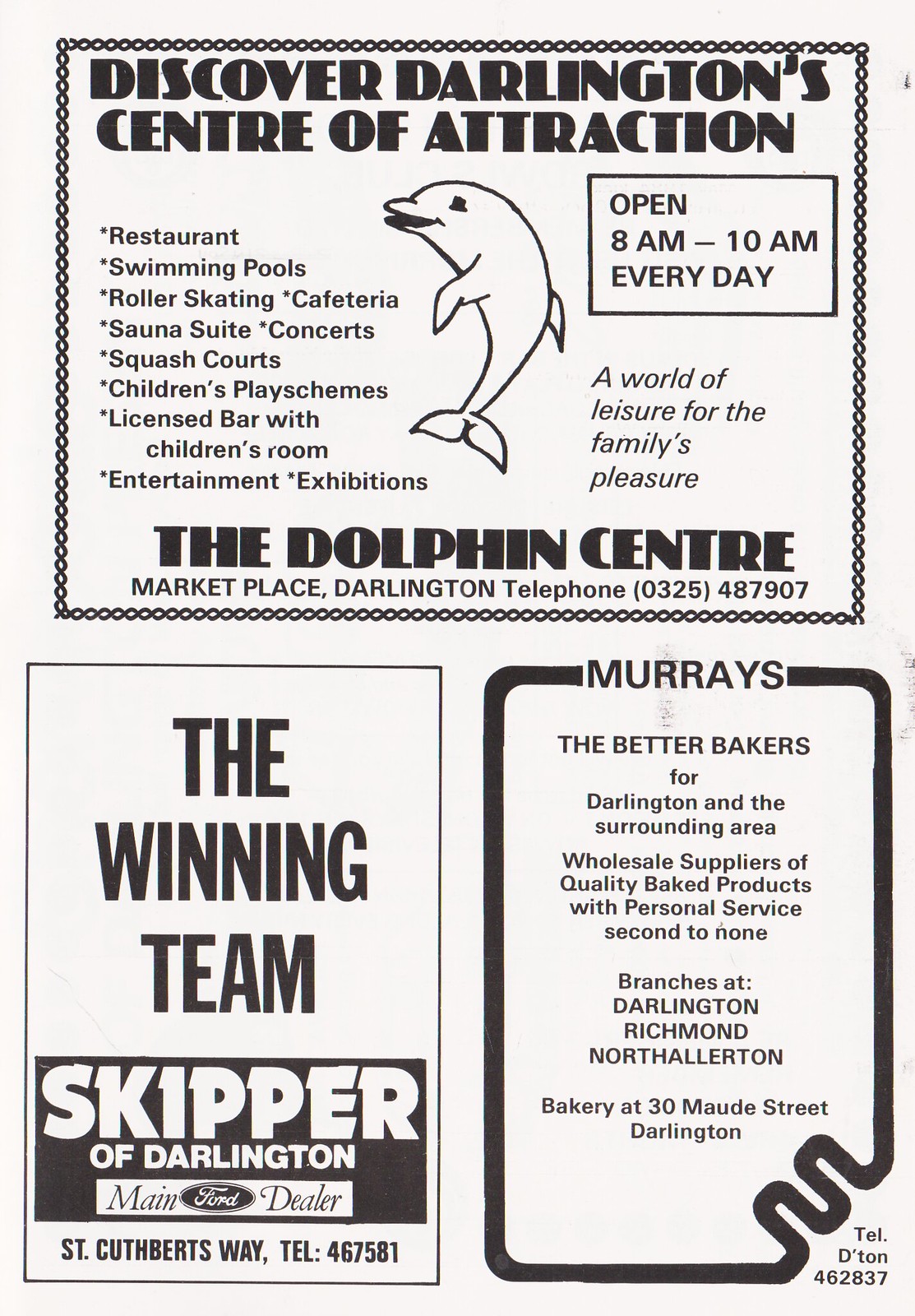The image features a black-and-white advertisement page, possibly from a program or newspaper, divided into three primary sections. The top section showcases an ad for the Dolphin Center, outlined with a decorative black chain-link border. The ad prominently features a dolphin illustration and the bold headline, "Discover Darlington Center of Attraction." Below, it lists various amenities such as a restaurant, swimming pools, roller skating, squash courts, children's play schemes, and a licensed bar with children's room entertainment and exhibitions. The ad emphasizes family leisure with the slogan, "A World of Leisure for the Family's Pleasure," and provides the operational hours from 8 a.m. to 10 p.m. daily, followed by the location and contact number for the Dolphin Center in Market Pet Lace, Darlington.

In the bottom left section, there is an advertisement for the Ford dealership in Darlington, known as "The Winning Team" and "Skipper of Darlington." It provides the address and phone number for the dealership at Cooperts Way, along with the contact number 467581.

The bottom right section features an ad for Murray's, described as "the better bakers for Darlington and the surrounding area." It highlights their reputation as wholesale suppliers of quality baked products with unmatched personal service. The ad lists various branches including those in Darlington, Richmond, and Allerton, specifically mentioning the bakery at 30 Magnet Road, Darlington, along with the phone number.

The entire page is white with black text, maintaining a consistent, monochromatic theme and featuring some black smudges on the right side near the top and middle.